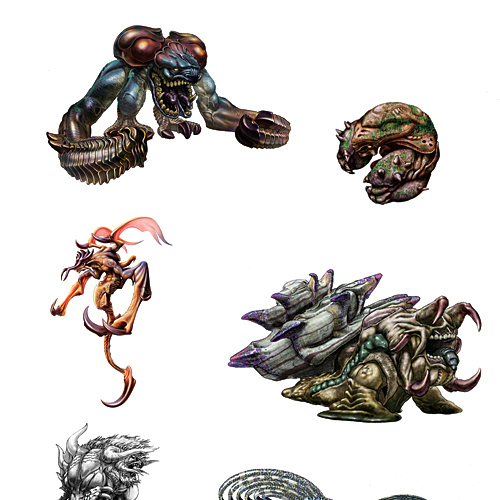The image features six dynamically designed, vividly colored creatures against a white background, resembling characters from action-packed games or movies, though they are somewhat eerie. The top left monster, characterized by massive arms, an open mouth brimming with sharp teeth, and two sturdy legs, is primarily colored in blue and brown. Adjacent to it on the top right is a small reptilian-like creature, snail-like in its features, with a brown and green palette. Directly below this is a peach-colored creature with long, leg-like appendages positioned upwards. To its right is a formidable creature with tortoise-like traits, identifiable by its open mouth lined with sharp edges and a rugged, sharp stone shell on its brown body.

In the bottom section of the image, partially cropped creatures add an element of mystery. One of them is a silver-toned figure with pinkish and yellow hues, noted for standing on one leg with long limbs and pink, flame-shaped ears. Another creature, with a bizarre configuration of six duck-like heads, showcases a complex blend of green, tan, and purple colors. The image's palette includes orange, pink, yellow, blue, green, tan, and silver, adding complexity and vibrancy to the diverse appearances of these fantastical creatures.